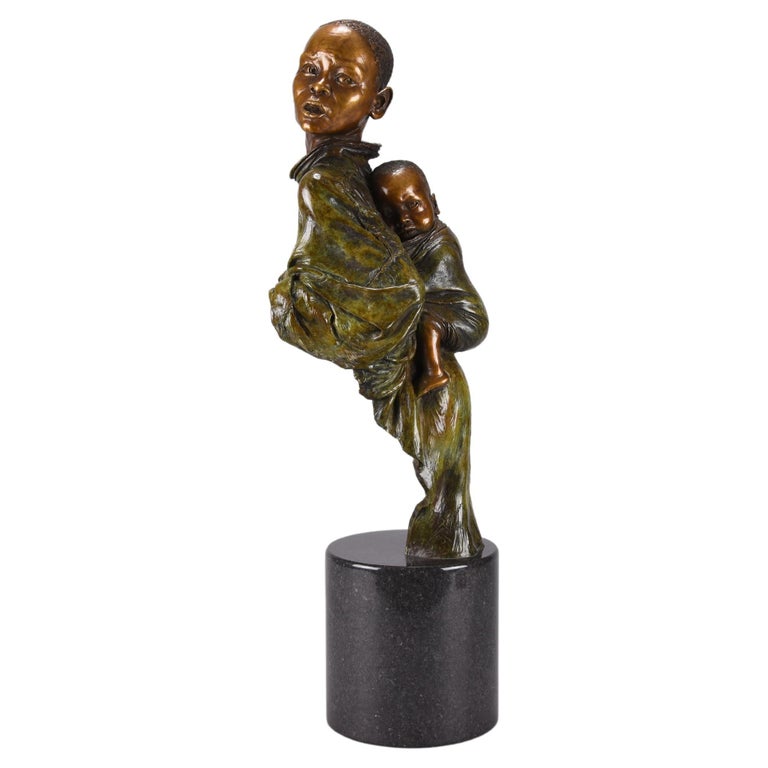The image showcases a detailed bronze statue of an African woman, accentuated with a goldish copper-toned face and subtle hair details. She carries a small baby strapped to her back under a swaddle blanket. Both figures exude expressions suggesting sorrow and hardship, with the mother looking slightly to the side with a frown and the baby also appearing hungry and unhappy. The woman's attire, a greenish copper long shirt, drapes around her form with a collar and displays an olive-brown hue under certain lights. This ensemble begins from a shiny, round, cylindrical pedestal resembling black marble. The statue, somewhat abstract yet evocative, powerfully captures the essence of maternal resilience and struggle.